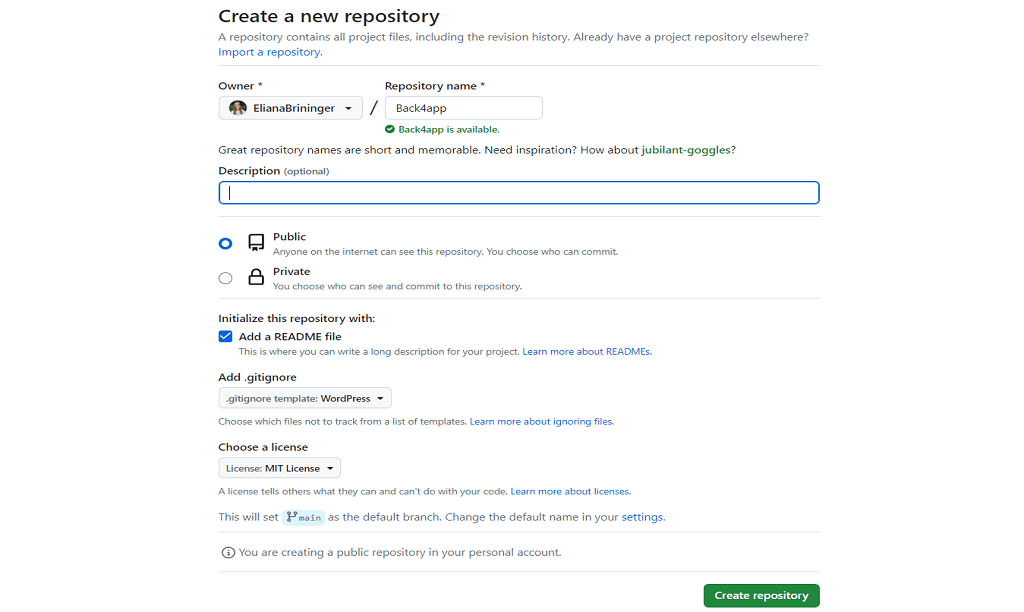The image captures a screenshot from a mobile device displaying a GitHub page for creating a new repository. At the top, the heading reads "Create a new repository," followed by an explanatory text: "A repository contains all project files, including the revision history. Already have a project repository elsewhere? Import a repository," with the "import a repository" phrase highlighted in blue for clickable action.

Below this, the owner of the repository is identified as "Eliana Brininger" with a star icon next to her name. The name of the repository is "Back 4 App," shown with a green confirmation message stating, "is available." A prompt beneath it suggests, "Great repository names are short and memorable. Need inspiration? How about Jubilant Googles?"

The description field is marked as optional. The visibility setting shows that "Public" is selected, indicated by a filled blue circle, while the "Private" option remains unselected. A checkbox is ticked next to "Add a README file" with the heading "Initialize this repository with." Below this, there is an option to add a ".gitignore" file. The page continues downward to a green button labeled "Create repository" at the bottom.